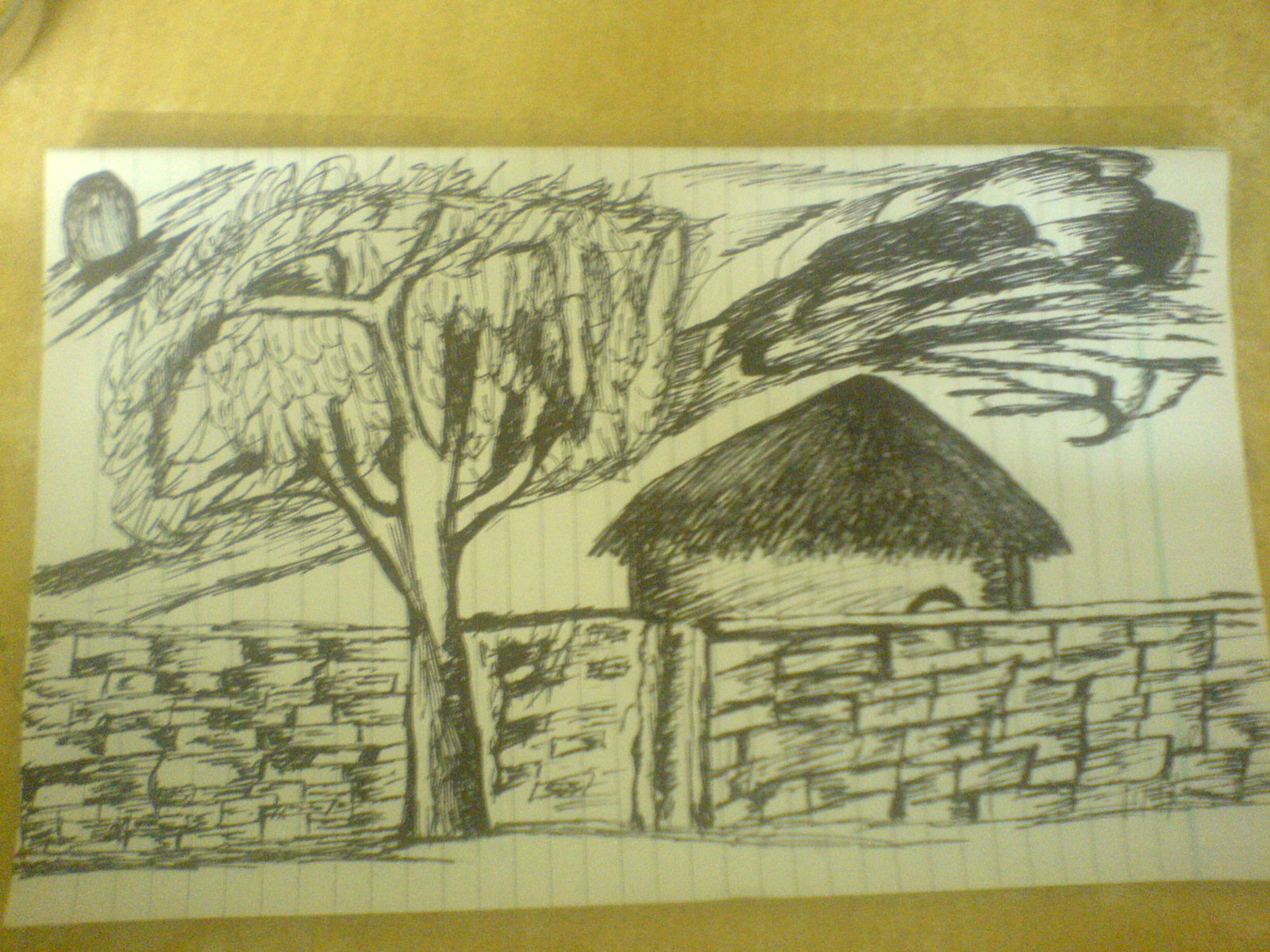A detailed hand-drawn charcoal sketch is depicted on a white sheet of paper, positioned in landscape mode. The sketch is notably rough and sketchy, adding to its rustic charm. The white paper is centrally mounted on a larger lime green rectangular sheet of paper, providing a vibrant and contrasting background which enhances the visibility of the artwork.

The artwork itself illustrates a quaint little thatched roundhouse, nestled behind a rustic woven wattle fence, exuding an aura of simplicity and traditional craftsmanship. In the foreground, a solitary tree stands with a curious lump perched at its top, which could be interpreted as either a bird or a nest, inviting viewers to ponder its identity.

Above the roundhouse, an ominous, heavily darkened cloud looms, contributing a dramatic and almost foreboding atmosphere to the scene. The stark contrast between the dark cloud and the lighter elements of the sketch intensifies the emotion conveyed through this detailed and expressive piece.